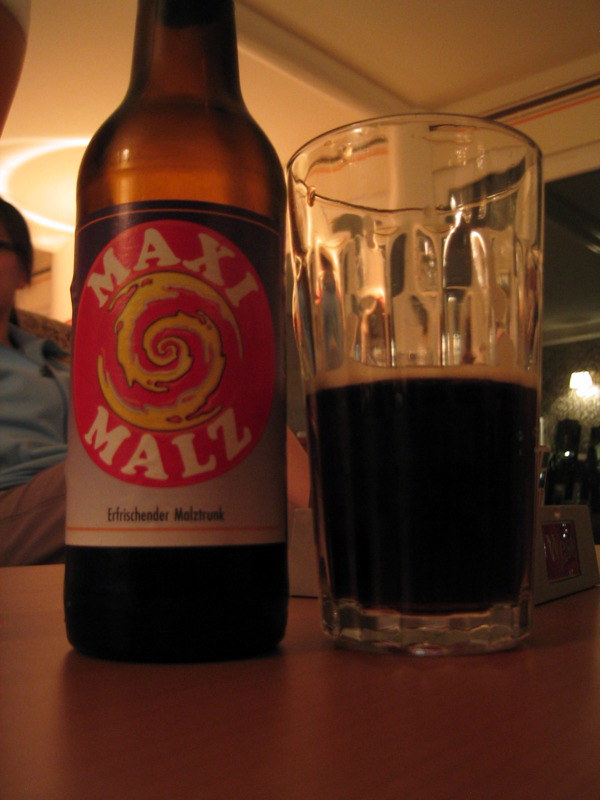In the dining room, a zoomed-in shot of a coffee table reveals intriguing details. On the left side of the table, there's a brown bottle with a label featuring a red circle with white text reading "Maximalz." Inside the circle, a striking yellow and black swirl draws attention. In the middle of the table, a glass is heavily filled with a dark beer, topped with a thin, small head of foam. Part of a person's face and body, wearing a blue shirt and grey pants, is visible on the left side of the image, lounging on a couch.